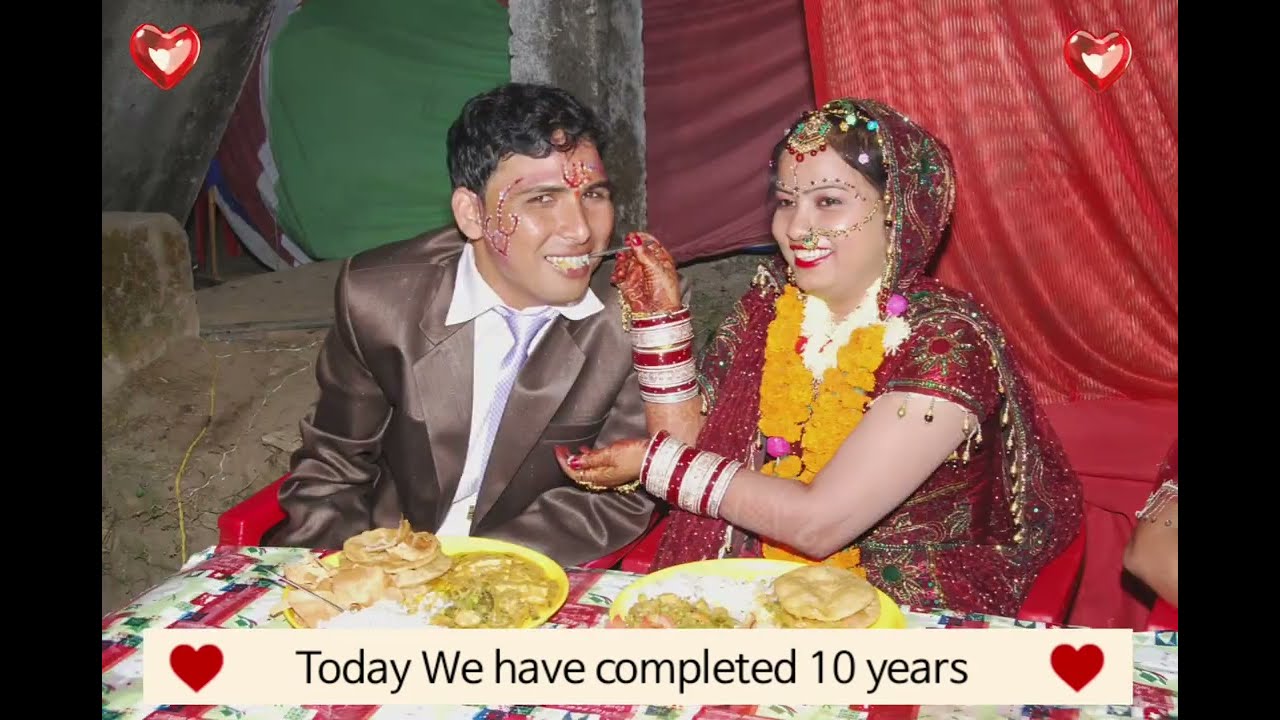This vibrant color photograph captures an Indian marriage celebration, showcasing a man and a woman seated at a table adorned with a gingham-patterned quilt. The couple is feeding each other, highlighting a moment of mutual affection and tradition. Behind them, red and green drapes create a festive backdrop, with a banner at the bottom that reads, "Today we have completed 10 years," flanked by red hearts. The floor to the left appears bare with a sprinkling of hay.

The man, with dark skin and short curly black hair, wears a shiny brown satin suit paired with a white dress shirt and a light lavender tie. Henna decorates his cheeks and the top of his forehead as he gazes at the camera, attempting to smile while taking a bite. The woman, adorned in a maroon outfit sparkling with gold and yellow accents, dons an impressive array of ornate jewelry. This includes red and white bangles, a nose ring connected by a chain under her scarf, and a head ornament resting on her forehead. Henna patterns outline her eyebrows. Despite feeding her husband, she gazes off into the crowd with a big smile, encapsulating the joy of the occasion. The table in front of them holds various plates of Indian food, including naan bread, served on bright yellow plates. The photograph not only captures their attire and setting but also the essence of their enduring bond.